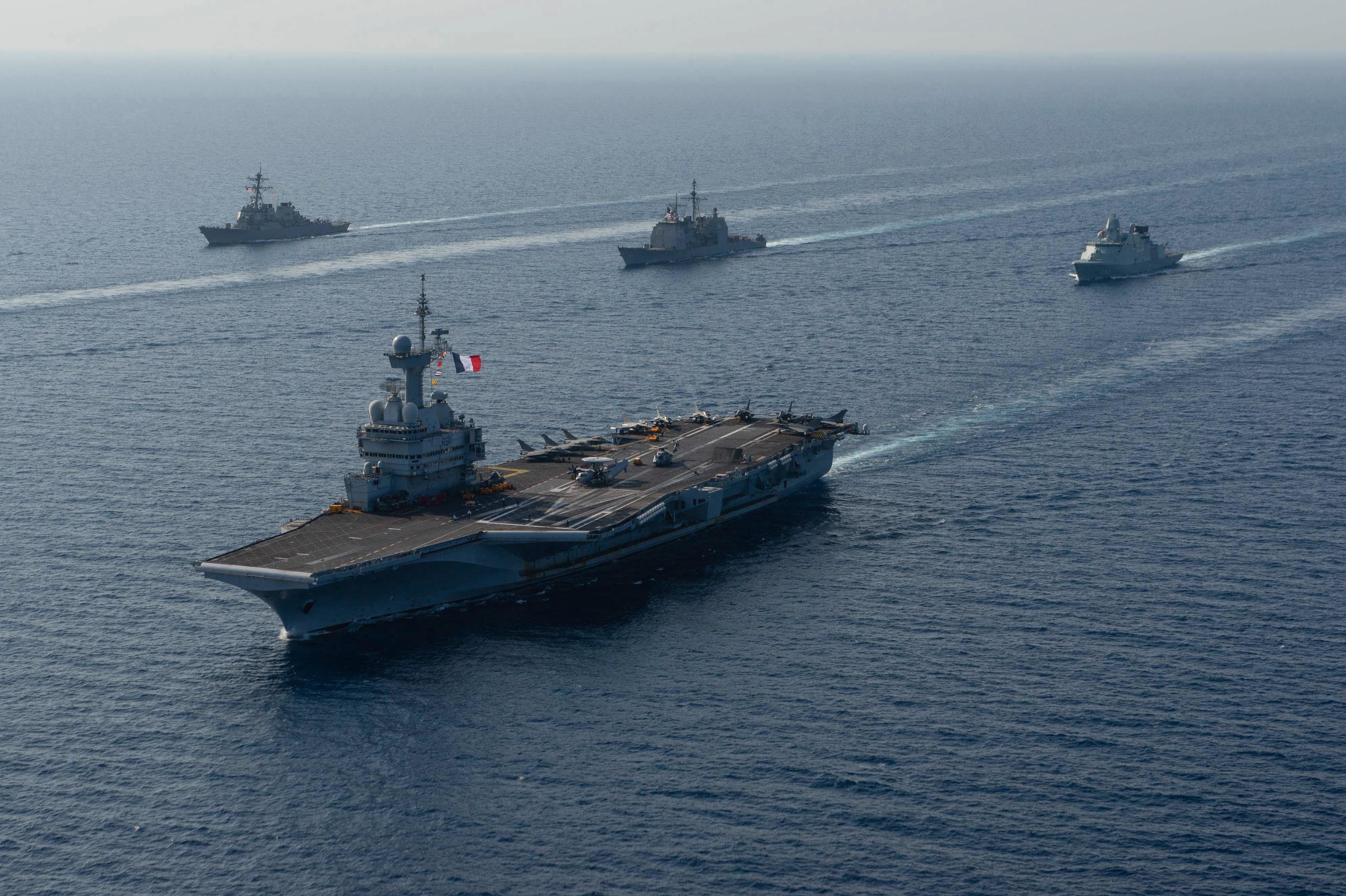In this detailed photograph, we see a large aircraft carrier prominently positioned in the foreground of the ocean scene. The carrier, flying a French flag from its control tower, which is located on the left side of the vessel, features what looks to be radar equipment. At least four or five aircraft are parked on its flat deck. The calm blue ocean spreads out beneath a light gray, hazy sky, with no significant waves disrupting the surface, just the normal ripples. Behind the aircraft carrier, and further back in the distance, three additional military ships can be spotted, each leaving a white trail in the water as they move forward. There's also an indication of the wake from a fifth, unseen ship. These ships are all heading toward the bottom left of the frame. At the very top of the picture, the horizon line distinctly separates the gray sky from the varying blues of the ocean.